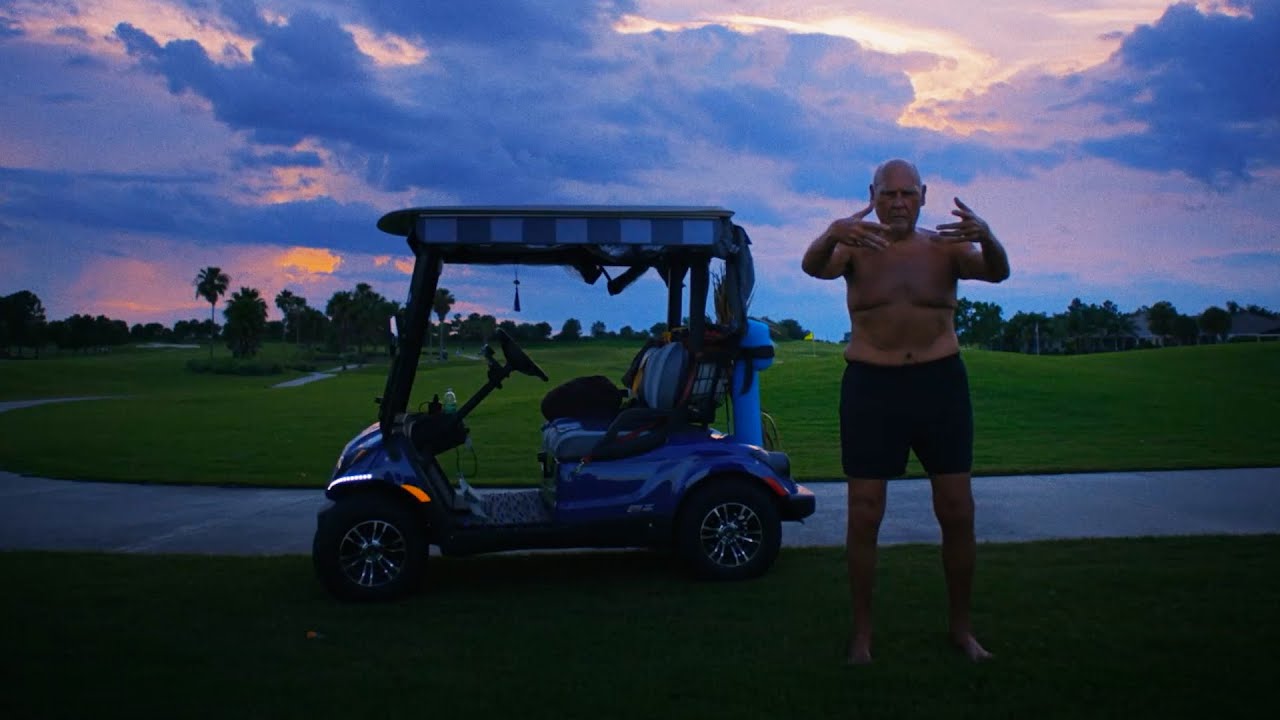In this photograph, a shirtless, elderly man stands next to a blue golf cart on a golf course. He is clad only in black shorts and possibly boxers, revealing a slightly overweight and flabby physique with notable love handles and a lighter tone around his belly compared to his mostly dark skin. The man is bald and performing a double-handed gesture, possibly an exercise or meditation pose, toward the camera. The scene is captured during twilight, under a dim and cloud-covered sky tinged with blue and subtle hues of orange. To his left, a striped-roofed blue golf cart is parked along the sidewalk. The well-maintained, closely shaven grass of the golf course stretches into the distance, bordered by green trees and a faintly visible church steeple. A pathway extends from behind the man, winding through the layout of the golf course.